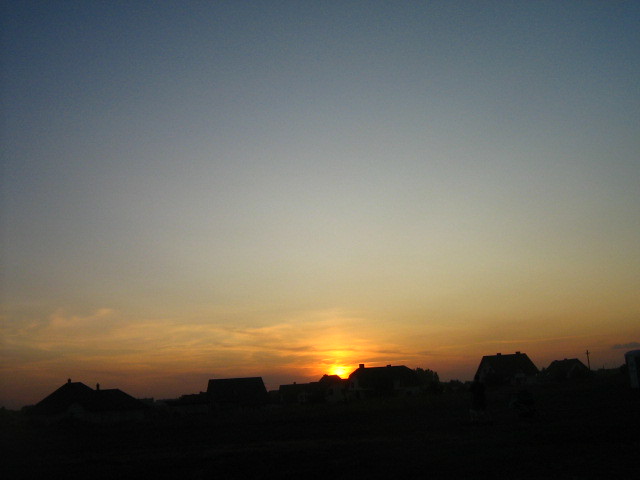This photograph captures a serene sunset over a silhouette of buildings on a hillside, viewed in landscape orientation. In the foreground, several blackened houses and buildings sit along the ridge of a slope, their details obscured by the brilliant light of the setting sun. One house's roofline is clearly outlined, complete with a distinguishable chimney. The sun, a vibrant yellow orb, is just above the roofline of one of these buildings, while bands of lavender and orange clouds streak across the lower part of the sky. Higher in the sky, the light transitions from orange to a gradient of twilight blues, growing darker towards the top. In the distance, trees add subtle depth to the scene. The clear sky lacks any stars, adding to the calm realism of this representational photograph. The image is neither dated nor signed.